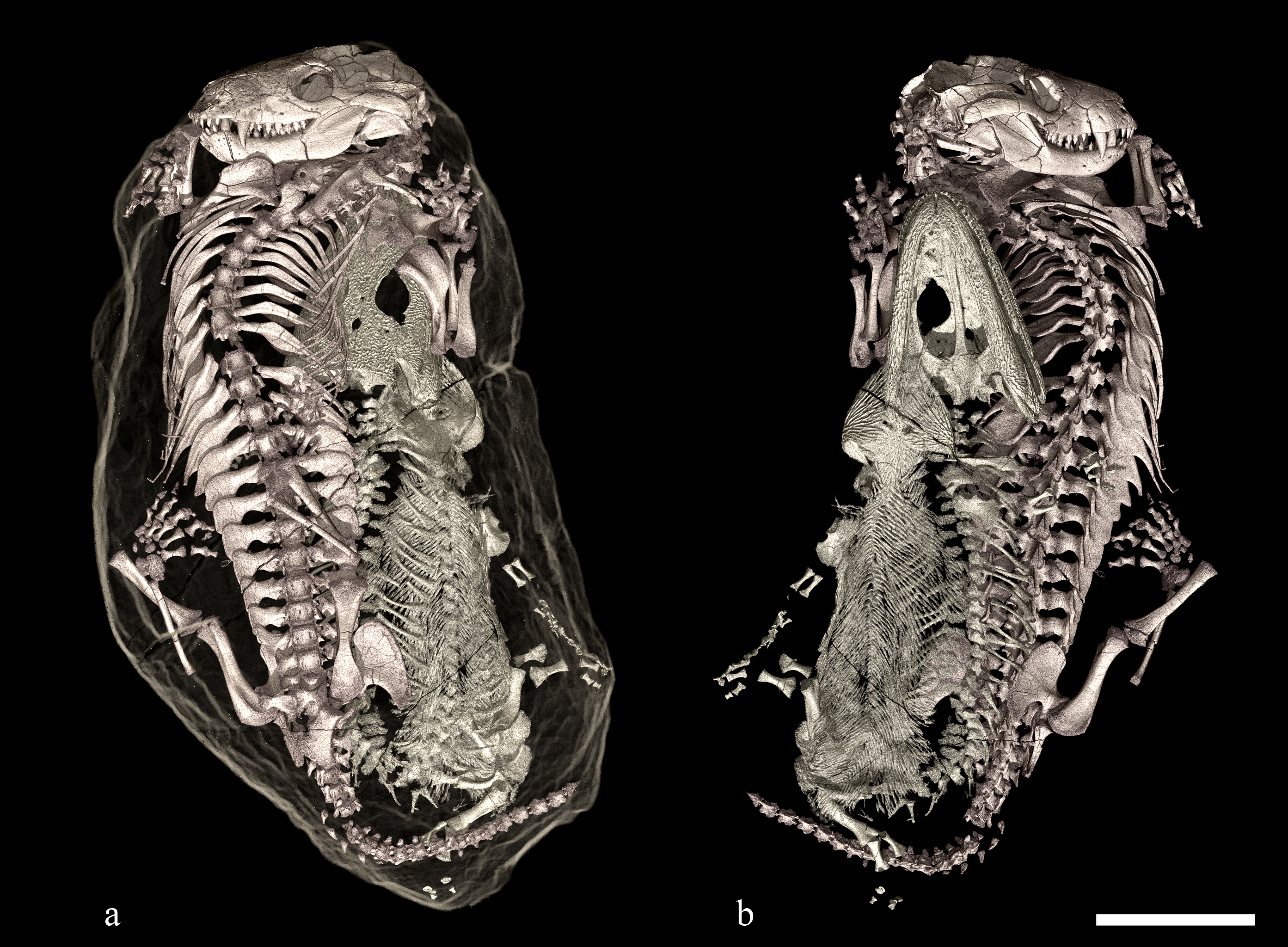This detailed black-and-white photograph features two highly similar skeletons, labeled A and B, against a stark black background. The skeleton on the left, marked as A, is oriented leftward, while the one on the right, labeled B, faces right. Both skeletons are in a curled, almost cocoon-like position. They have flat, elongated skulls reminiscent of alligators, complete with sharp, jagged teeth on the upper jaws. The bodies of these creatures are characterized by full ribcages extending down to narrow tails, and the legs vary in size with smaller front legs and larger back legs. Noteworthy is the presence of additional skeletal elements and scales surrounding the main figures, suggesting some parts might be dislodged. Overall, these skeletons exhibit a prehistoric, reptilian appearance, potentially shrinking down versions of larger creatures like dinosaurs or large lizards.